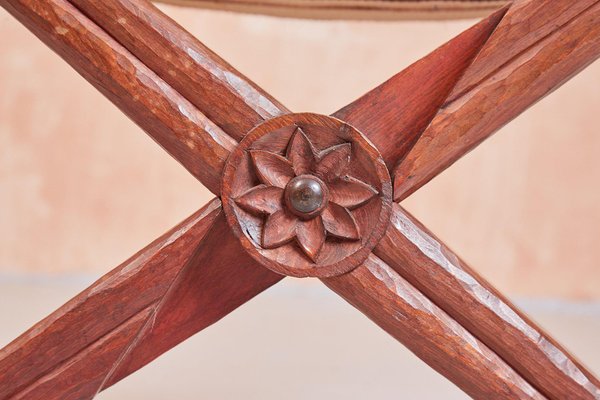This detailed photograph showcases a meticulously handcrafted wooden structure, possibly part of a piece of folding furniture like a chair or table. The foreground features two diagonal wooden crossbars arranged in an X pattern. These crossbars appear smooth, having been carefully whittled and sanded. Where they intersect is a central, round section, intricately carved to resemble a lotus flower with eight pointed petals. The flower carving features a circular core, which appears to have a bolt running through it, holding the structure together. The wood is a rich reddish-brown hue and exudes the quality of skilled craftsmanship, likely done with both hand tools and power tools. The background of the image is blurred, displaying an orange or pink hue that further highlights the exquisite details of the wooden piece.